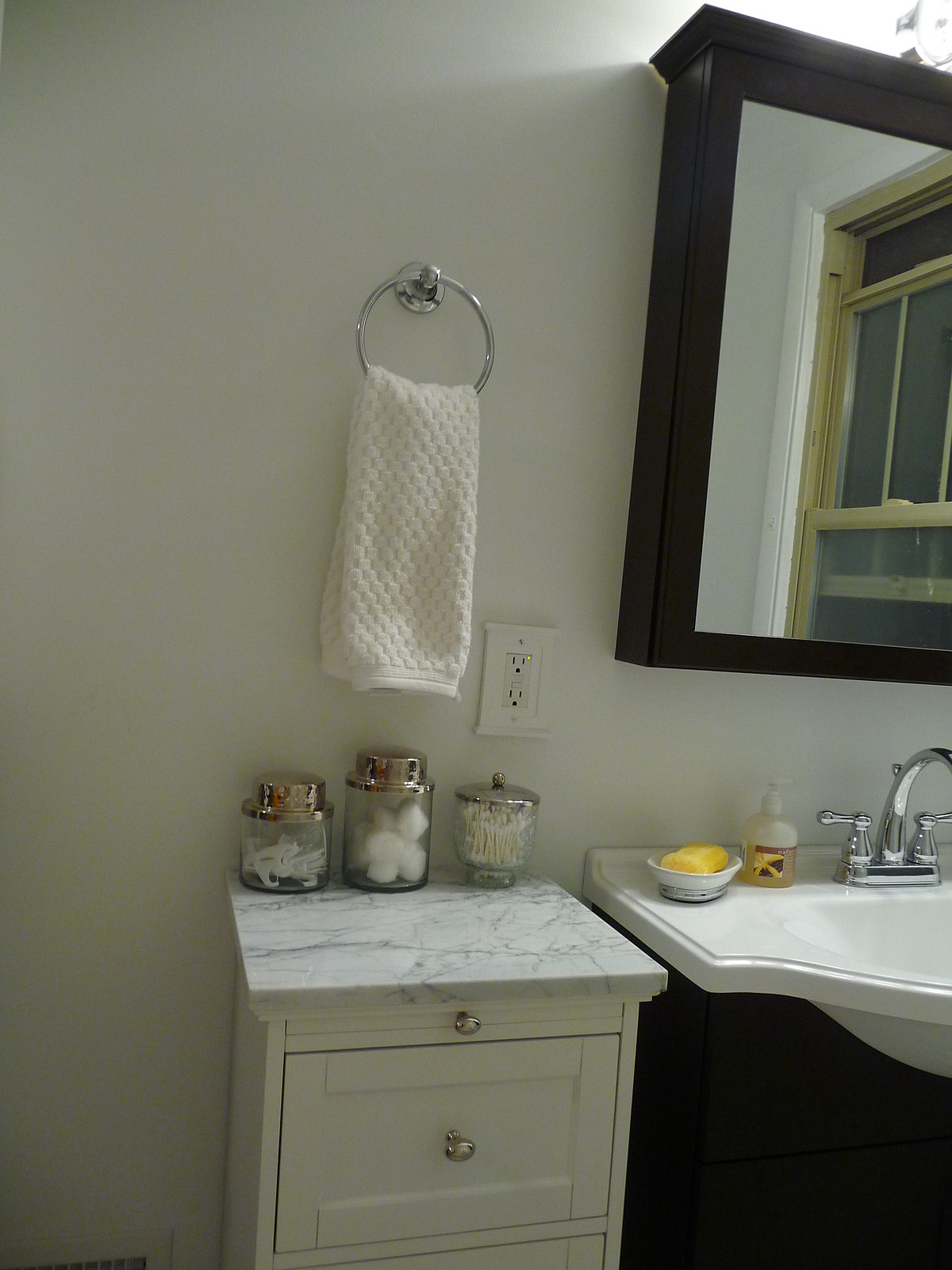In the top-right corner, a black-framed mirror reflects a closed window, revealing a night-time scene outside. The window's glass shows a divided pane structure with brown framing and white trim. Below the mirror, a white porcelain sink is neatly organized. A white dish on the left holds a yellow soap bar, while to the right, there is a pump bottle of liquid soap adorned with a floral label. The faucet, featuring a silver handle on both sides, each with a thin bar that can be twisted, sits centrally.

To the left of the sink, a fuzzy white towel hangs from a silver ring. Below it, the white granite countertop with interwoven black lines supports three jars, each with a silver lid. One jar is filled with an unidentified substance, another with cotton balls, and the last with Q-tips. The countertop flows into cabinetry below, comprising a small and larger drawer, each with a silver knob.

Towards the left of the image, an outfit, square in shape with small lights at the top resembling two holes, is visible. Above the entire setup, a light source subtly illuminates the scene, giving it a cozy ambiance.